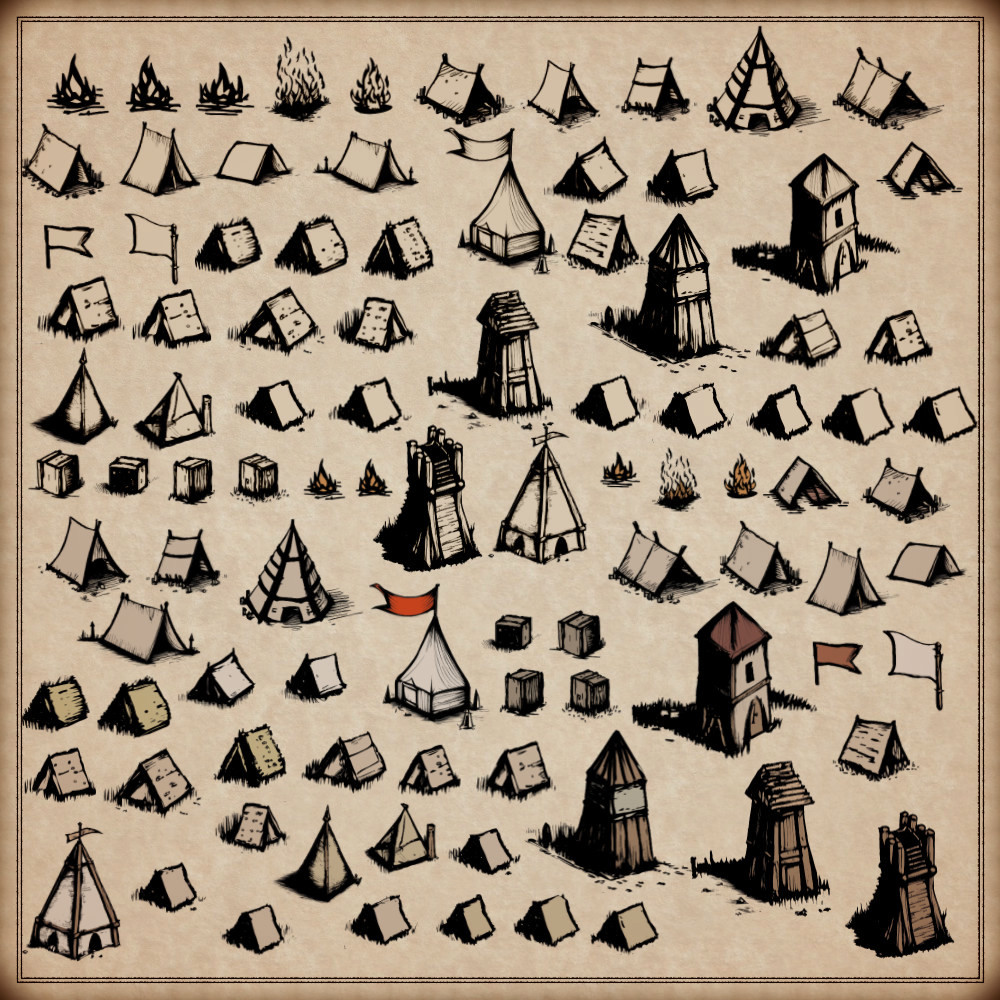The image illustrates a medieval campsite bustling with a variety of small, canvas tents and taller, wooden huts. The setup appears like a military encampment or ancient village. Scattered throughout are several flags, with a notable red flag flying above a central, white tent. The entire scene, depicted in meticulous black sketches on a tan or light gray backdrop, contains about fifty elements, including lookout towers and campfires situated in the upper left and center parts of the image. This intricate drawing, possibly sourced from a textbook or history book, vividly captures the essence of historical camping arrangements.